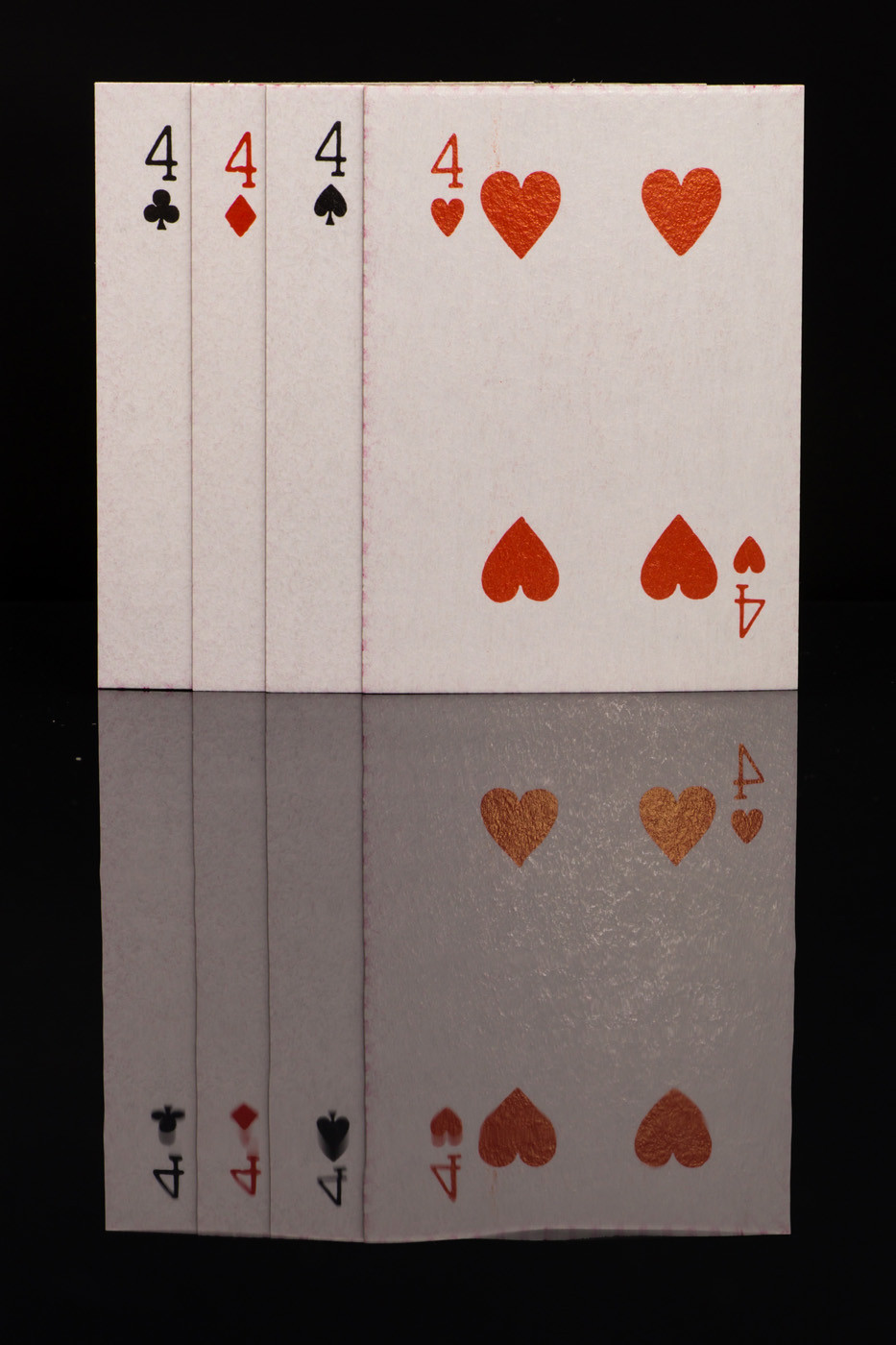This image features a set of four playing cards meticulously arranged against a stark black background. The cards themselves boast crisp white faces adorned with either red or black symbols and text, indicative of their respective suits. From left to right, the cards displayed are the four of clubs, four of diamonds, four of spades, and four of hearts, each partially overlapping the next in sequence. This cascading arrangement results in the four of hearts prominently sitting atop the stack, clearly showcasing its quartet of heart symbols. Beneath it, only the upper left corners of the other cards are visible, each marked with their corresponding number "4" and suit icon.

Intriguingly, the lower half of the image mirrors the top, with a slight variation—the card reflections rest on a gray-toned background instead of pure white. This reflection flawlessly maintains the alignment and order of the cards above, serving as a symmetrical counterpart. The alignment is precise with both the top and bottom edges of the cards perfectly horizontal and the sides vertically parallel, creating a visually striking composition.